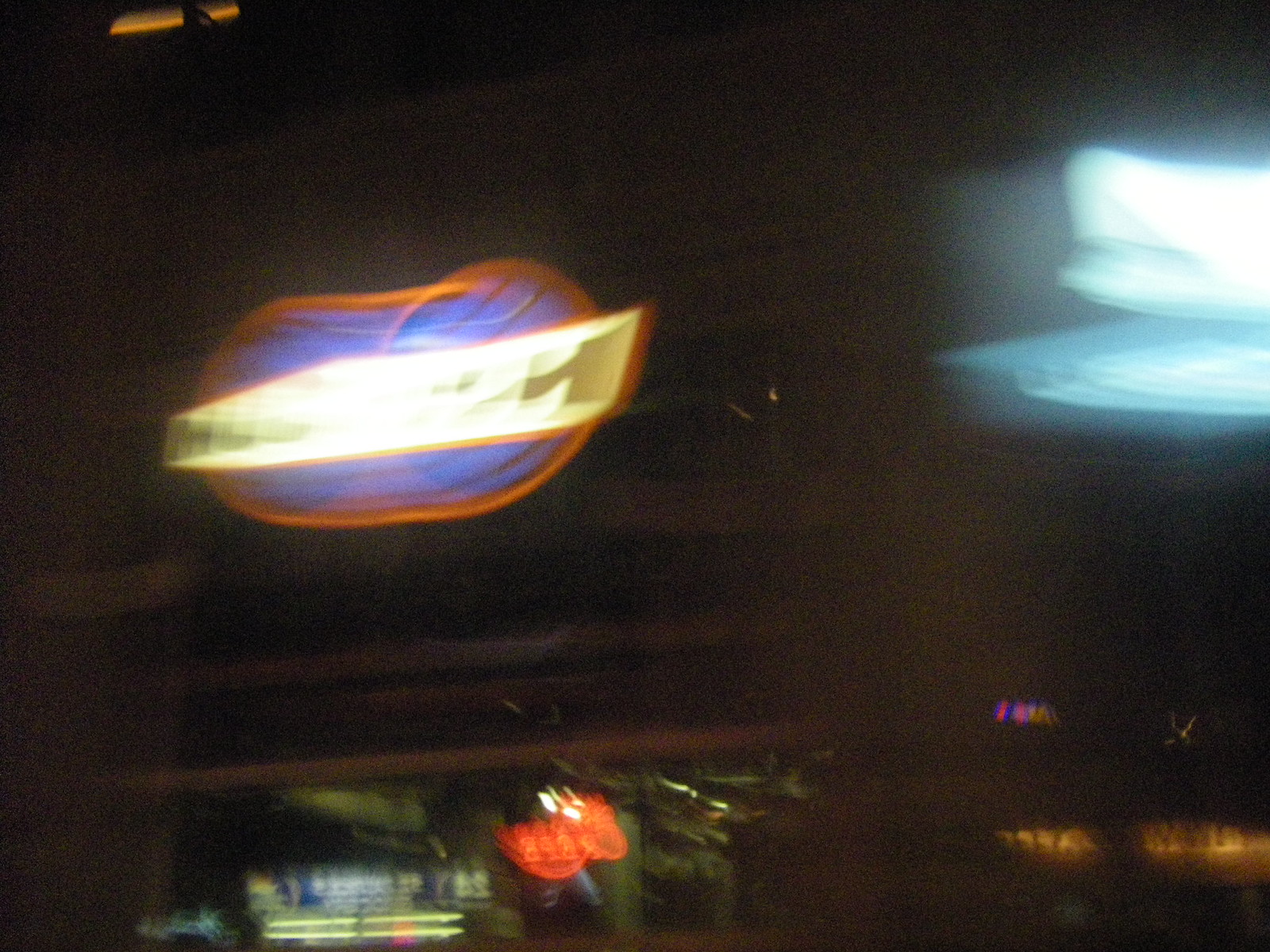A blurry photograph of a nighttime outdoor scene. The image features a prominent yet indistinct neon sign near the center left, emitting a red or orange glow with a bright white section in its center. To the right, a vivid blue light stands out against the dark backdrop. At the bottom, several windows are faintly visible alongside additional neon signs, one glowing red and another white, contributing to the vibrant nighttime ambiance.